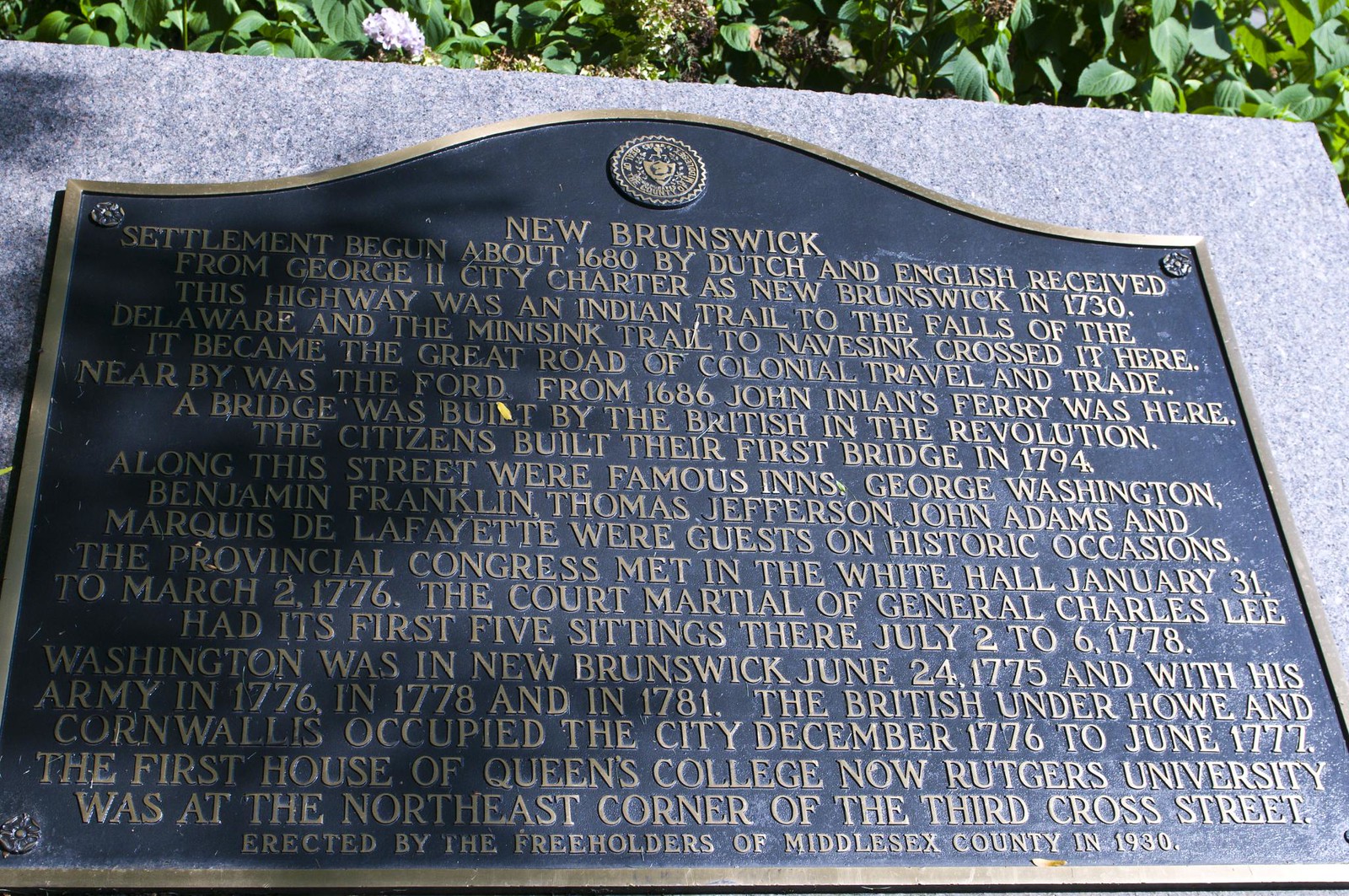The image depicts a historical plaque mounted on a piece of granite or marble, showcasing a scene with an off-white to black and red speckled background. The plaque itself is black with a gold outline and a distinctively rounded top, featuring a circular insignia or crest at the center. The text on the plaque is written in gold font and provides a detailed history of New Brunswick: "New Brunswick, settlement begun around 1680 by Dutch and English, received from George II, city charter as New Brunswick in 1730. This highway was an Indian trail to the Falls of the Delaware, and the Menesink Trail to Navesink crossed it here. It became the great road of colonial travel and trade. Nearby was the ford from 1686. John Inyans Ferry was here. A bridge was built by the British in the Revolution, and the citizens built their first bridge in 1794. Along this street were famous inns; George Washington, Benjamin Franklin, Thomas Jefferson, John Adams, and Marquis de Lafayette were guests on historic occasions. The Provincial Congress met in the White Hall from January 31st to March 2nd, 1776. The court-martial of General Charles Lee had its first five sittings there, July 2nd to 6th, 1778. Washington was in New Brunswick on June 24th, 1775, and with his army in 1776, 1778, and 1781. The British under Howe and Cornwallis occupied the city from December 1776 to June 1777. The first house of Queen's College, now Rutgers University, was at the northeast corner of the Third Cross Street, erected by the freeholders of Middlesex County in 1930." The setting includes leaves, grass, and a single violet-purple flower near the top left, with light shining from the right side, casting a shadow to the left.